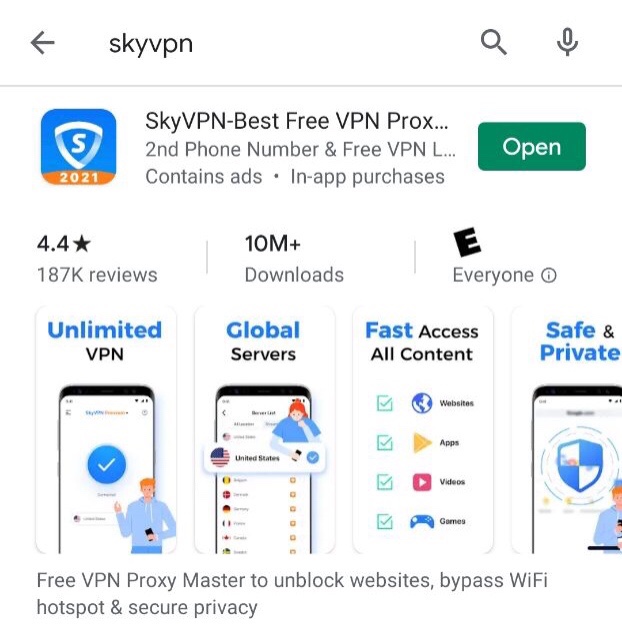Here’s a cleaned-up and detailed descriptive caption for the image:

---

The image showcases the Play Store interface with a white background. The search bar at the top contains the query "Sky VPN." Below the search bar, the selected app is prominently displayed. The app is named "Sky VPN - Best Free VPN Proxy, Second Phone Number, and Free VPN" and indicates that it contains ads and offers in-app purchases. The app icon, located to the left of the app name, is blue and features a white "S" symbol, with a sheet-like design in white. Additionally, "2021" is written in white on an orange background within the icon, signifying the app's relevance for the year 2021.

On the right side of the app listing, there is a green "Open" button, indicating that the app is already installed. The app boasts a rating of 4.4 stars from 187K reviews, with over 10 million downloads and is marked as suitable for everyone.

Below the app information, four sections describe the app’s features, displayed in a combination of blue and black text. The sections are as follows:

1. Unlimited VPN
2. Global Safest
3. Fast Access to Internet, Websites, Apps, Video Apps, Games
4. Safe and Private Browsing

Finally, the app description further elaborates on its capabilities: "Free VPN proxy master to unblock websites, bypass Wi-Fi hotspots, and secure privacy."

---